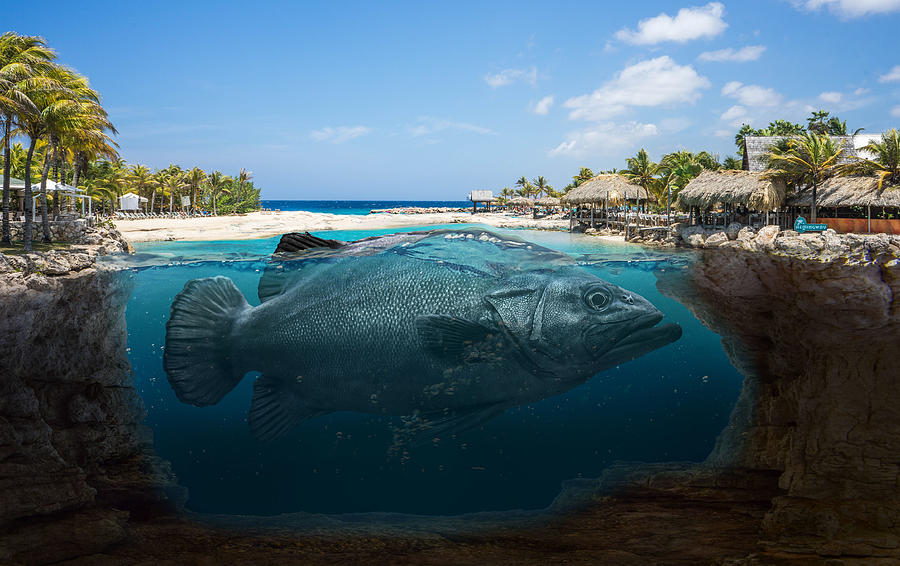This highly detailed and striking image, likely digitally altered, portrays a serene tropical lagoon framed by a quaint island village. The village, characterized by thatched huts, more modern buildings, and lush palm trees, is visible on both the left and right sides of the image. The photograph captures a cross-sectional view of the lagoon, revealing the entirety of the underwater scene along with the surface landscape. 

At the center of the image lies the lagoon, where a massive, silvery-gray fish dominates the water, occupying roughly 80% of the visible underwater space. The fish's head faces the right, while its tail stretches toward the left, its mouth partially open and an expressionless look on its face. The fish's body protrudes slightly above the water, creating a dramatic focal point. The water in the lagoon transitions from a bright, clear blue near the surface to a darker, almost black hue toward the bottom, enhancing the depth and mystery of the scene.

In the background, beyond a sandy beach and a small sandbank, the tranquil ocean extends to the horizon under a beautiful blue sky dotted with a few clouds on the right. The overall mood of the image is peaceful yet intriguing, capturing both the beauty of a tropical paradise and the surreal presence of an oversized fish within a picturesque lagoon.